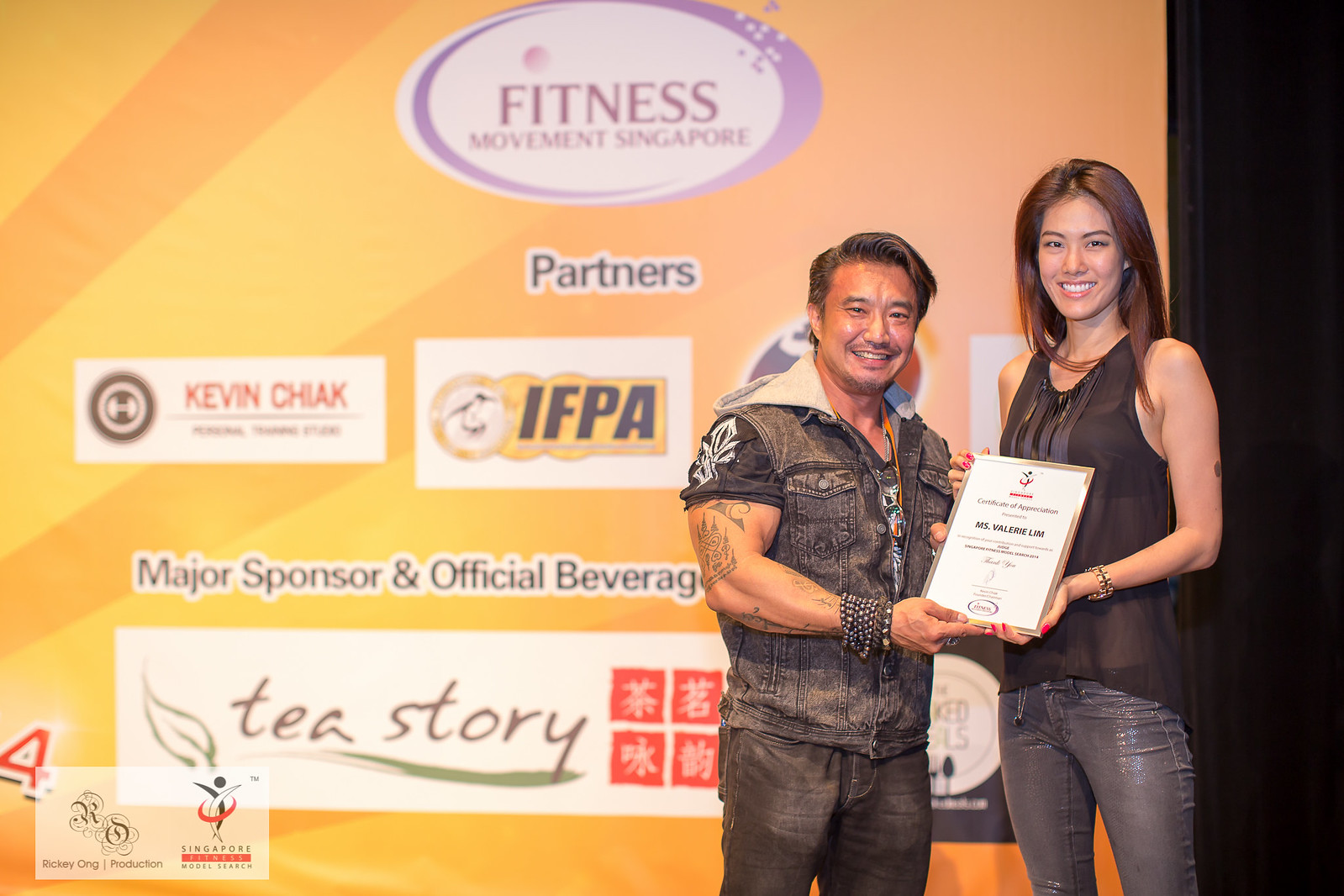This indoor photograph captures a dynamic stage scene, viewed from the right-hand corner. The rectangular image, wider than tall, features a backdrop of black curtains on the right side and a projection screen on the left. Beams of yellow and orange light emanate from the lower left, transitioning into orange as they move across to the right side. Centered before the backdrop, a man and a woman, both of Asian descent, are engaged in a moment of recognition.

The man, shorter and of muscular build with notable biceps, is of older age and has Asian features. He dons a black jean leather vest with a gray hood, layered over a black shirt, and pairs this with gray-blue jeans. His right wrist is adorned with multiple bands. He extends an award that reads "Certificate of Appreciation, Ms. Valerie Lim" to the woman beside him. The woman, about a head taller, has center-parted dyed brown hair and is smiling directly at the camera. She wears a sheer black sleeveless blouse over a black bra and shiny, skinny blue jeans.

Behind them, a large banner with an orange background and various advertisements is displayed. The banner reads "Fitness Movement Singapore Partners Kevin Chia, IFPA, Major Sponsor and Official Beverage, Tea Story." The bottom left corner includes a smaller superimposed section with symbols, stating "Ricky Orrick Productions Singapore Model Search." The scene vividly captures a moment of recognition and celebration, enhanced by the vivid lighting and detailed attire of the individuals.